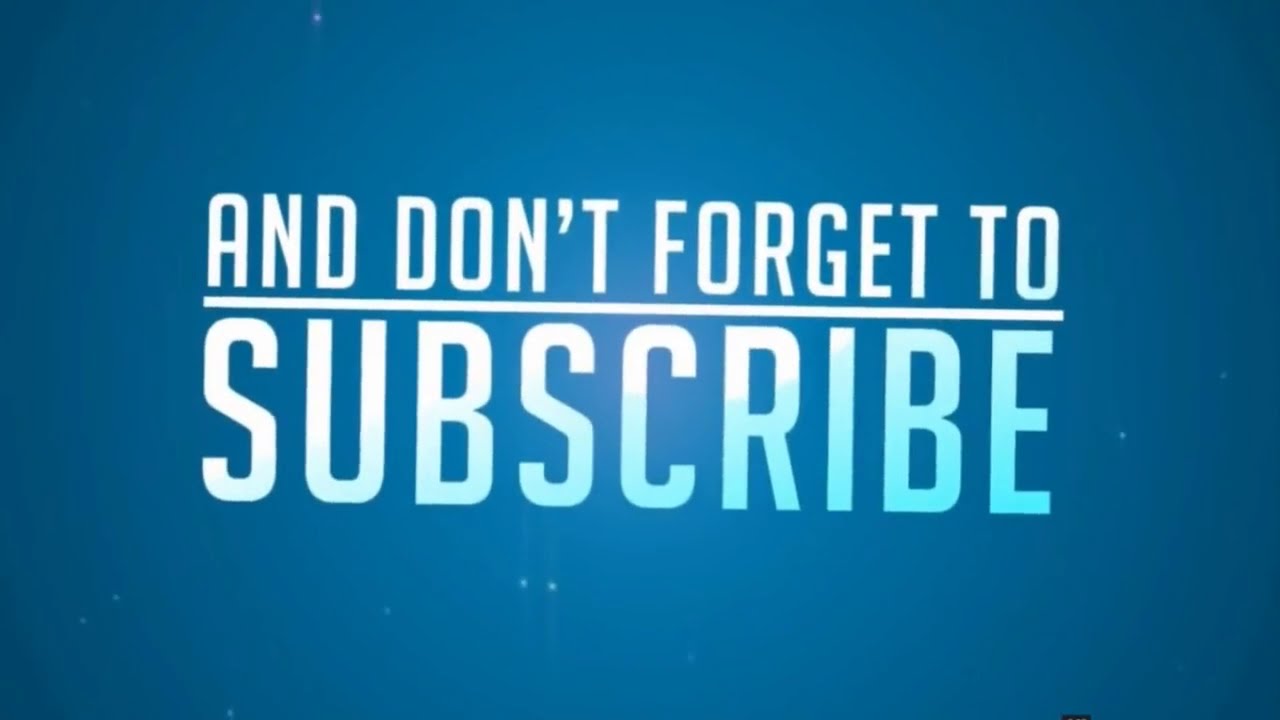The image features a vivid blue background with a subtle gradient that transitions from a lighter blue at the center to a darker blue along the edges. Scattered across the background are faint white dots, adding texture and depth. Anchoring the center of the image are two lines of white text in capital letters. The top line reads "AND DON'T FORGET TO" and is fully underlined. Below this, in larger letters that subtly fade into the blue background, the word "SUBSCRIBE" stands out. The design mimics the proportions of a high-definition TV screen, specifically a 1080p widescreen format, making it visually akin to a typical YouTube video prompt.